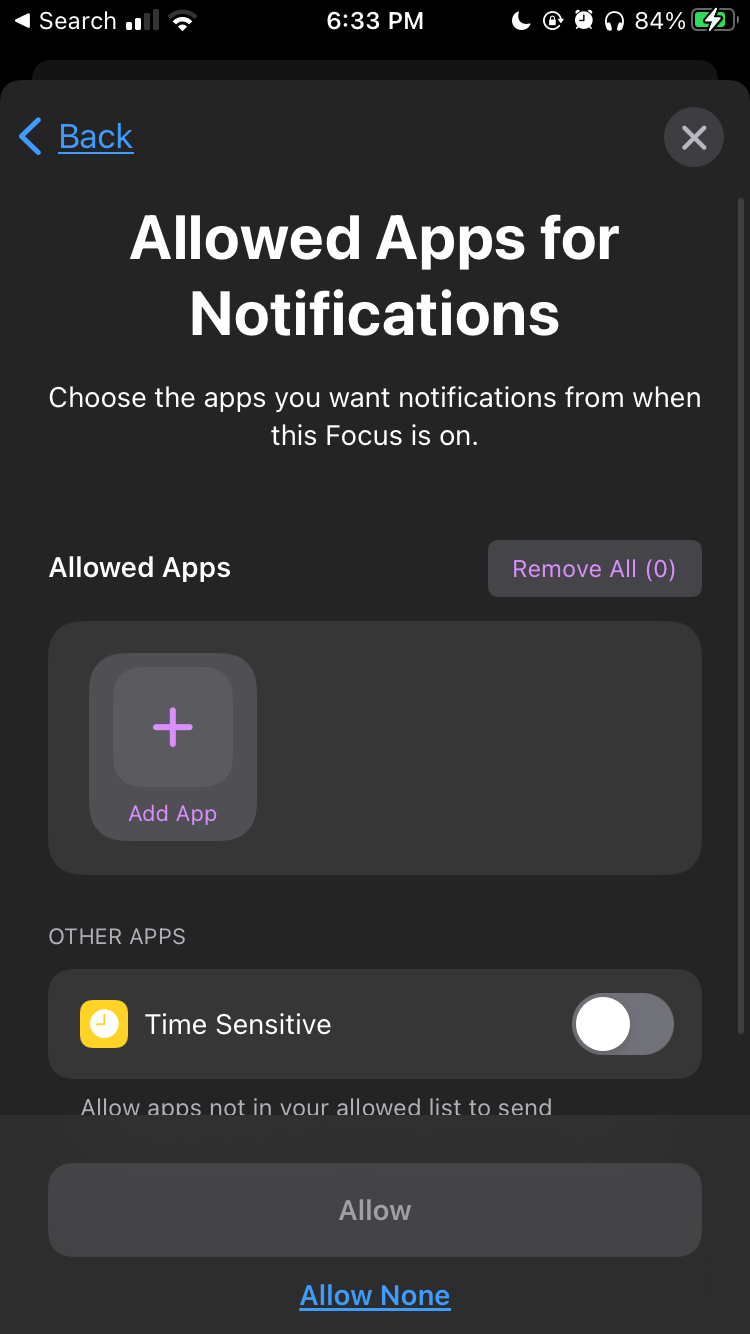The image described is a screenshot of a smartphone interface with a variety of elements displayed on a dark theme. 

At the top, a black background features the status bar elements. In the top left corner, white text displays "Search" next to a white left-pointing triangle icon. Adjacent to this are Wi-Fi signal bars, a pie-shaped battery icon, and a battery percentage indicator reading "84%", which is green with a lightning bolt symbol inside, indicating that it is charging. The time "6:33 p.m." is prominently shown in the center. On the top right, additional icons include a crescent moon (likely the Do Not Disturb mode), and a pair of headphones. 

Beneath the status bar, a section with a gray background shows navigation elements. In blue font, an underlined "Back" arrow points to the left, indicating a back button. To the right of this, a gray circle houses a white 'X' emblem.

Below that, in the main content area, white text reads "Allowed apps for notifications". In a smaller font, it advises, "Choose the apps you want notifications for when this focus is on." Directly below, a subtitle "Allowed Apps" is followed by a gray square containing purple text "Remove All [0]". Beneath this is another gray square with an interior gray circle containing a purple plus sign, indicating an option to "Add App."

Further down, a dark gray section is titled "Other Apps" in white font, featuring another gray square with a yellow square inside and an illustrated clock marking "Time Sensitive." This icon is followed by a toggle switch, depicted as a white circle on a gray background, currently in the off position.

At the bottom, a black background section displays a prompt in white font: "Allow apps not in your allowed list to send notifications." Below this is a gray button labeled "Allow" in the center. The final line in blue, underlined font reads "Allow None."

This detailed hierarchy of elements indicates it is likely a settings menu, guiding users to manage notification permissions for various apps in different modes or focuses.